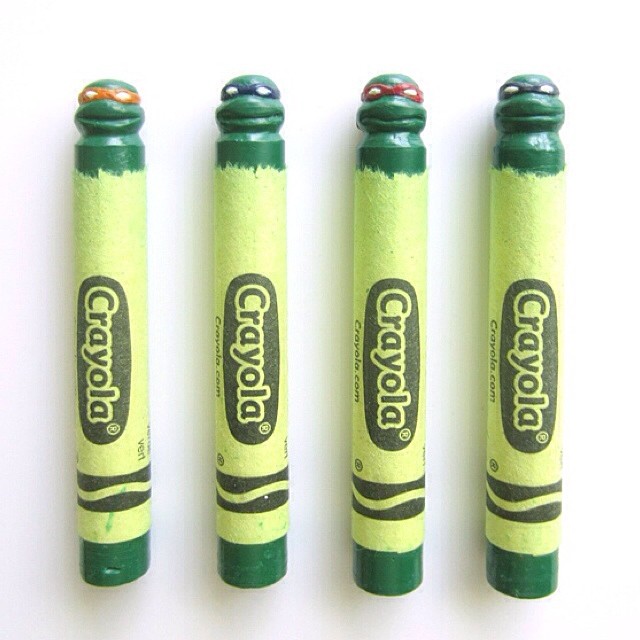The photograph features four dark green Crayola crayons arranged vertically against a white background with slight shadowing at the bottom. Each crayon has a yellow Crayola wrapper with the signature black wave and logo. Uniquely, the tips of the crayons are carved into the grinning faces of the Teenage Mutant Ninja Turtles, each sporting their iconic colored masks: orange on the left, followed by blue, then red, and lastly purple on the right. The intricate carvings and vivid colors give the crayons the appearance of turtle figurines with distinctive goggles, adding a playful and artistic twist to the traditional school supply.